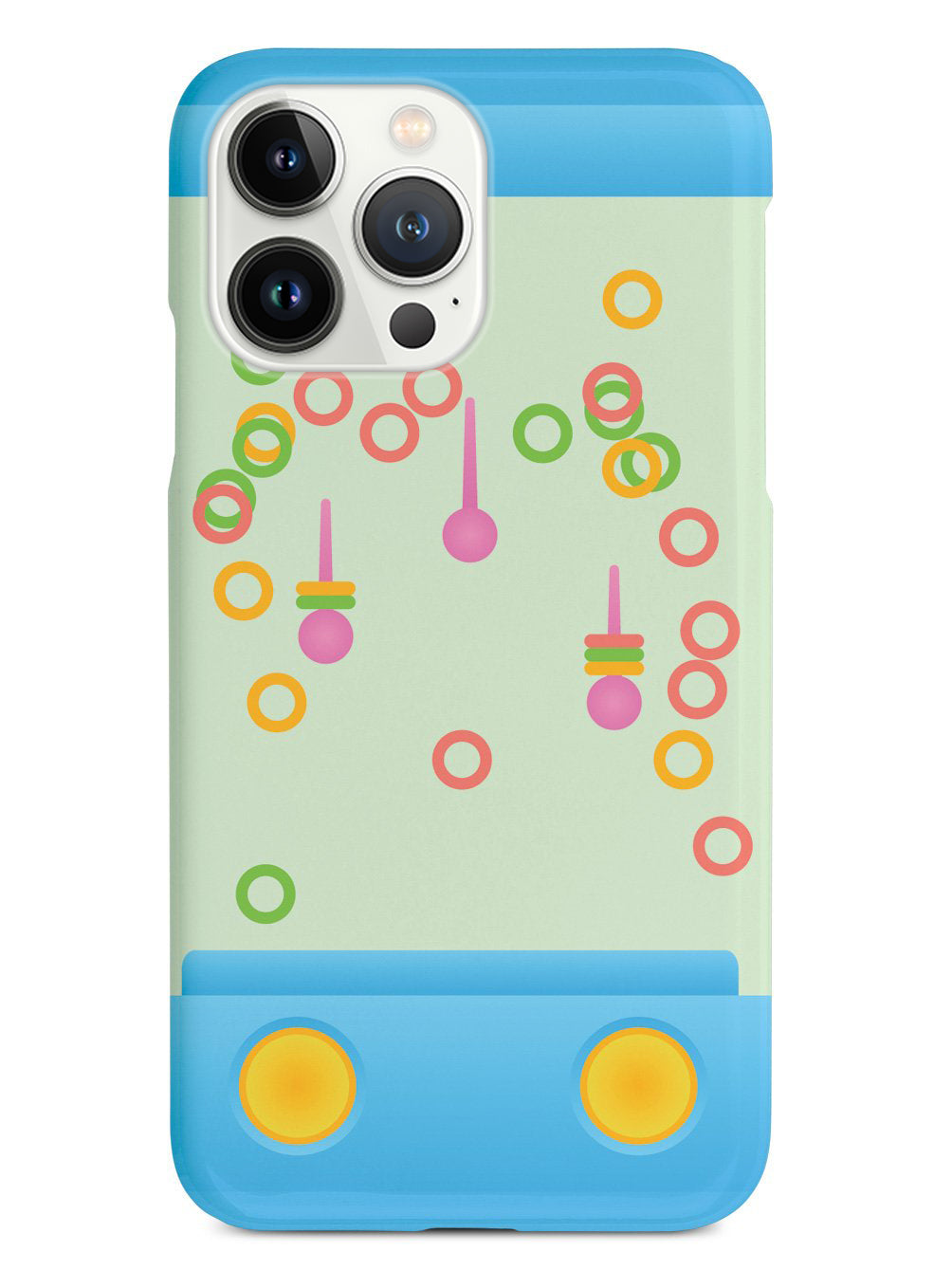This image depicts the back of a modern iPhone encased in a protective cover. The iPhone features the characteristic three-camera system in the top left corner. The case itself is colorful and vibrant with a cartoonish design. The top and bottom sections of the case are blue, while the central portion is a faded beige-green. Strewn across the middle of the case are multicolored rings in shades of orange, yellow, green, and pink, designed to appear as if they are cascading downward. These rings look like they are meant to land on small pink pegs, reminiscent of a classic ring-toss game. Two larger orange circles are positioned near the bottom of the case, flanking the charging port. The overall background of the image is white, highlighting the playful and vivid design of the iPhone cover.